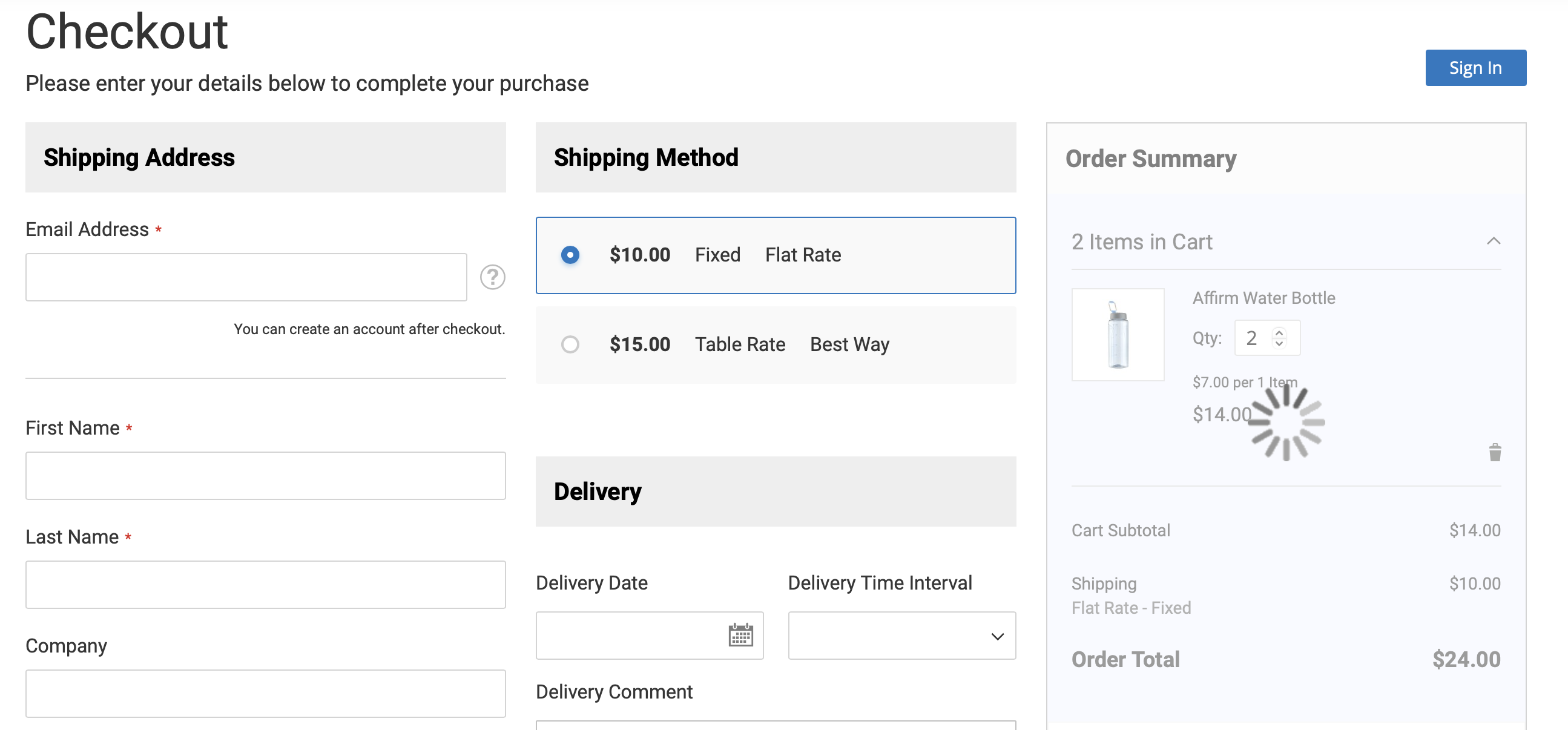The image features a detailed section of a checkout page. In the top left corner, bold black text reads "Check Out" with a large font size, and just below, in smaller letters, it says "Please enter your details below to complete your purchase." On the far right top corner, a dark blue rectangle with white text invites users to "Sign In."

Beneath the "Check Out" heading, a light gray rectangle displays the words "Shipping Address" in black letters. Below this section, the background transitions to white, featuring various form fields with black text.

The first form field is labeled "Email Address," marked with a red asterisk to denote a required field. To the right of this field outline, there is a small circle containing a question mark. Below, a note states, "You can create an account after checkout." 

A gray dividing line separates this from the next set of fields, which include "First Name" and "Last Name," both also accompanied by red asterisks. Each label has a corresponding gray-outlined rectangular input box.